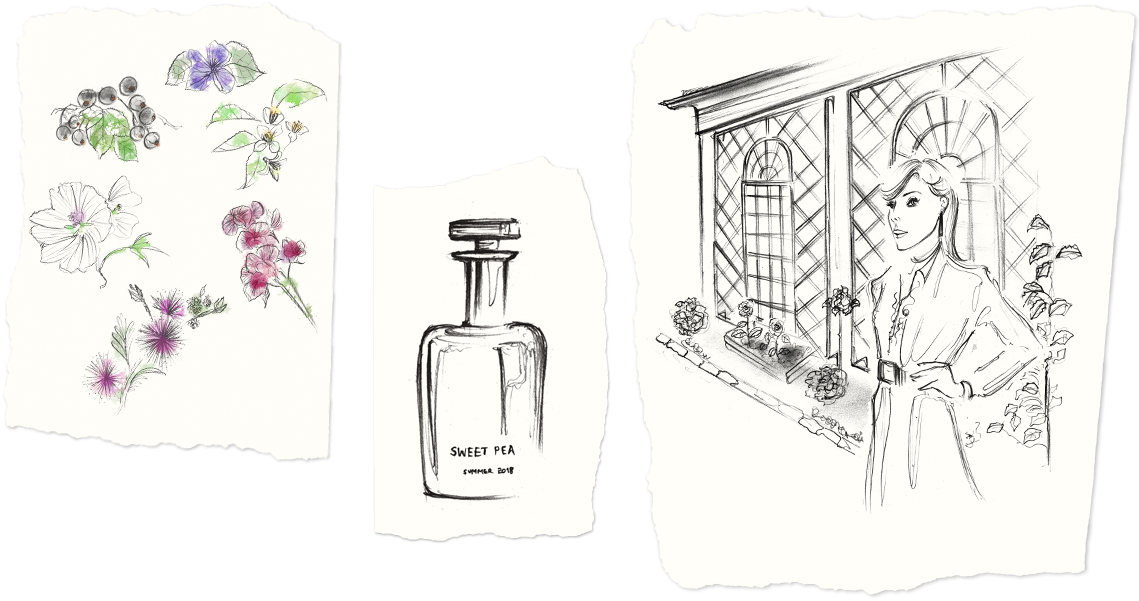The image consists of three separate, torn pieces of antique off-white paper, each featuring a detailed sketch. The leftmost paper depicts six colorful botanical drawings arranged in a circular pattern, showcasing various flowers and berries in shades of purple, dark red, white, and green, with elements like blueberries and petunias. The center paper displays a black and white pencil drawing of a rectangular perfume bottle labeled "Sweet Pea," capped with a simple stopper, and some unreadable text below. The rightmost paper features a black and white sketch of a woman in a cinched dress with a belt, standing outside an old-style building with large arched windows and surrounded by plants. The woman, adorned with a flower in her hair, has her hand on her hip and glances to the side, capturing a sense of timeless elegance.